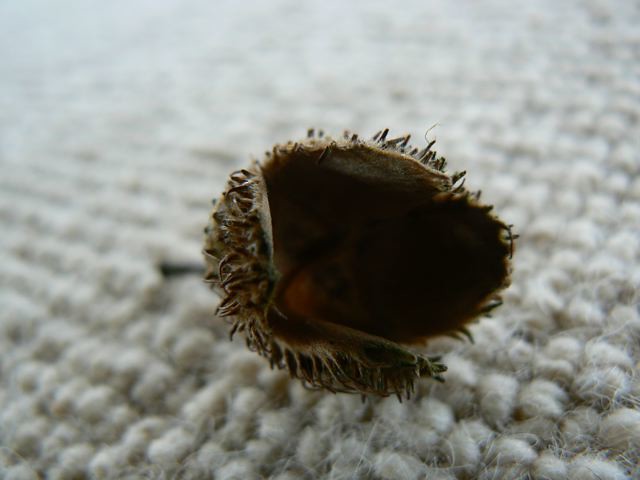The image showcases the spiky, brown, outer shell of what appears to be a seed or nut pod, possibly a chestnut pod, that has fallen from a tree. The shell is dark brown with a slight reddish tint and is covered in numerous spikes, giving it a prickly appearance. It is open and empty, revealing a dark hollow inside. The open shell, about the size of an acorn, is positioned facing to the right. The surface it rests on is a beige carpet with visible threads, likely a soft wool or natural fiber rug. The detailed texture of both the spiky shell and the woven carpet emphasizes a contrast between the shell's harsh exterior and the carpet's soft, woven nature. Care is needed around the shell as it looks like it could be painful to touch.